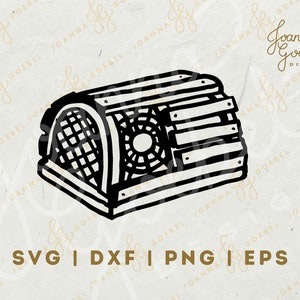The illustration showcases a meticulously crafted vector graphic in black and white, executed with pen-like precision. Central to the artwork is a semi-circular, tubular object reminiscent of an old-school 1920s or 1930s radio, constructed from multiple wooden planks. It features a rectangular base, above which lies a curved top adorned with intricate black mesh lines, suggestive of cross-hatched grating. Adding to its vintage charm is a section with a spiderweb pattern, creating an impression of shattered glass or an actual cobweb. This drawing masterfully utilizes varying line thickness to depict shadowing and depth, particularly noticeable on the top edge and the left side of the object, giving a dimensional quality to the wooden planks. Beneath the object, gold text lists the available file formats: SVG, DXF, PNG, and EPS. The entire artwork sits against an off-white background, subtly enhancing its black-and-white contrast. A cursive, gold-font inscription reading "Joanne" is visible in the top right corner and stretches diagonally across the image, adding a personalized touch to the intricate design.